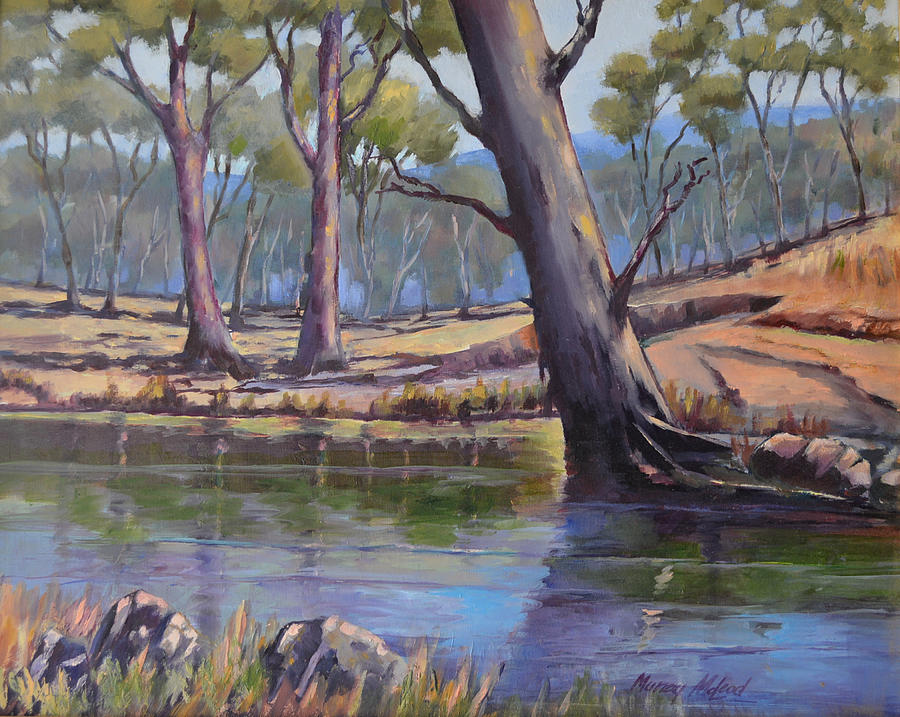This watercolor painting by Murray MacLeod depicts a serene creek or river meandering through a vibrant forest landscape. In the foreground, the shore is adorned with gray and black rocks, mingling with green and yellow grasses. The water itself is a blend of blues and greens, perhaps hinting at the presence of algae or reflections. A large, strikingly dark tree with bare branches leans over the river, its roots exposed and sprawling along the bank, suggesting it may be dead or dying. Floating sycamore leaves can be seen drifting on the surface, adding a touch of natural detail.

Beyond the creek, a dense array of trees with lush green foliage stand resilient, backed by rolling hills of brown earth and grassy patches. Above, blue mountains rise in the distance, creating depth and perspective. The painting, though not hyper-realistic, skillfully captures the essence of the natural scene, merging fauvist and impressionistic elements with its dynamic use of peaches, yellows, blues, and greens. The overall palette enhances the idyllic yet slightly melancholic atmosphere of this tranquil wilderness.